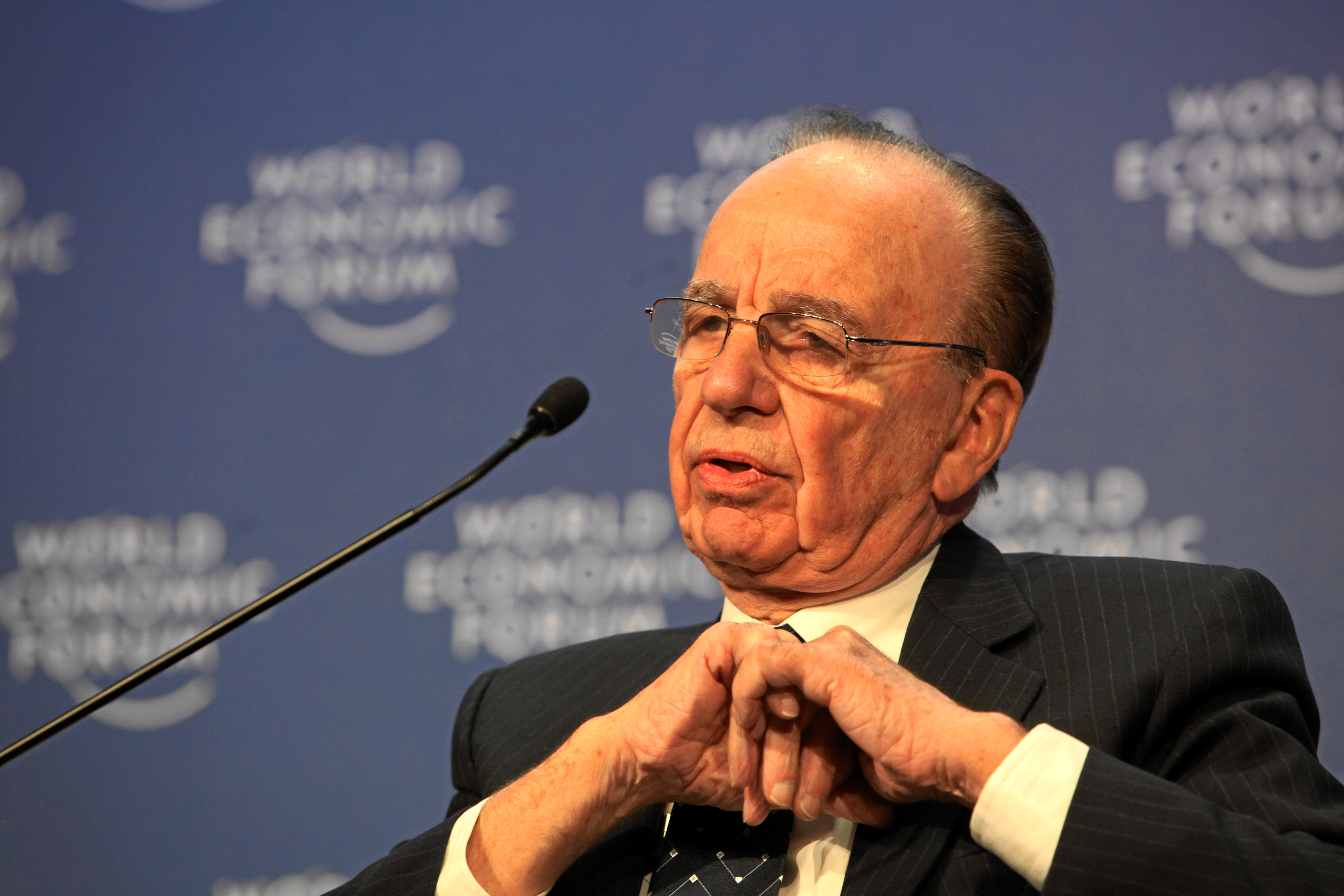In this photograph, an elderly European man in his 60s or 70s is situated in the left center of the image, addressing the World Economic Forum. He is wearing a black and white pinstripe suit with a white dress shirt and a blue tie featuring a geometric design. His receding hairline and glasses, along with the wrinkle lines on his face, suggest his advanced age. The man has slicked-back hair and sits with his hands clasped in front of him, his expression serious as he speaks into a small, skinny black microphone emerging from the side of the frame. The background features a cobalt blue wall with the repeated white lettering "World Economic Forum" and its logo, although this is slightly out of focus.